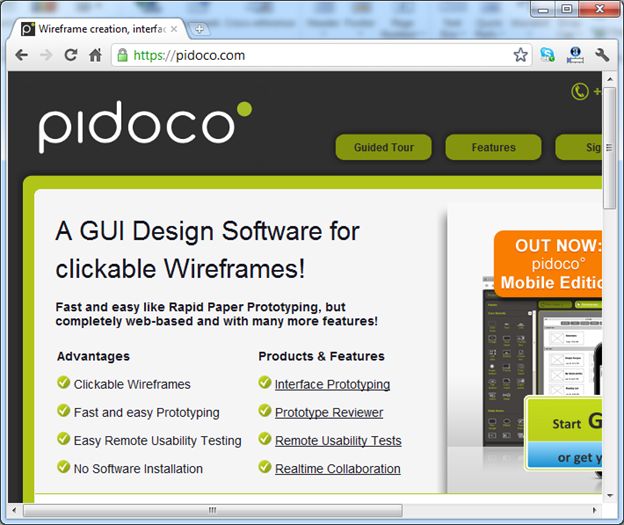The image displays a partially visible web page titled "Wireframe Creation Interface - PIDOCO." Due to the limited screen size, only a portion of the page is viewable, with some content appearing cut off. At the top of the page, a couple of tabs are visible, labeled "Guided Tour of Features." Further down, a section describes PIDOCO as a "GUI Design Software for Clickable Wireframes," emphasizing its capabilities for fast and easy prototyping similar to rapid paper prototyping but entirely web-based with additional features. The advantages highlighted include "Clickable Wireframes," "Fast and Easy Prototyping," "Easy Remote Usability Testing," and "No Software Installation." Additional sections visible in the image list various product features such as "Interface Prototyping," "Prototype Reviewer," "Remote Usability Tests," and "Real-Time Collaboration." Despite these detailed descriptions, the complete content of the web page cannot be seen in the depicted view.